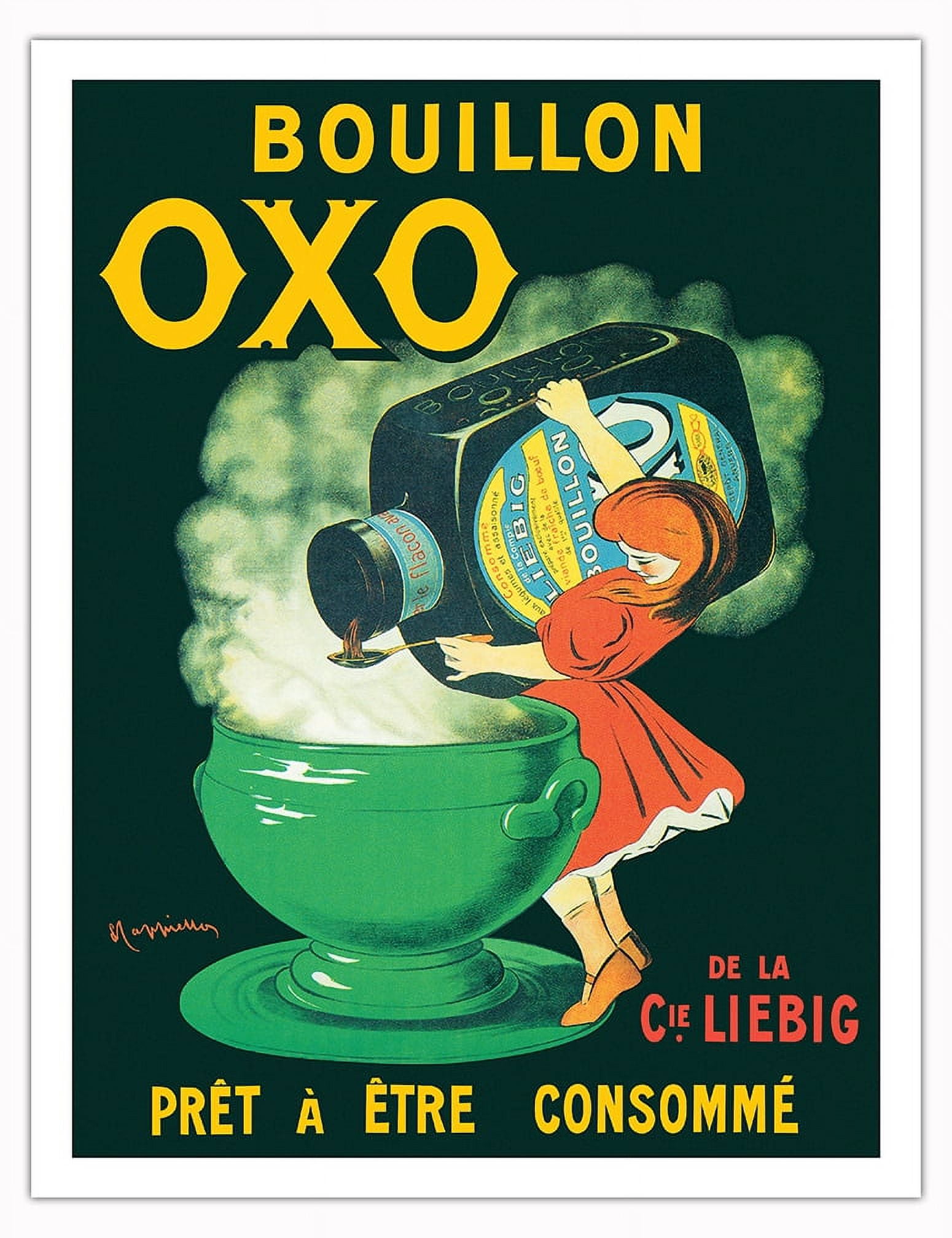This detailed vintage advertisement, likely from the early 20th century, features a stylized illustration with a black background. Central to the poster is a very small girl with striking red hair, dressed in a red dress with white petticoats and brown Mary Janes. She is holding an enormous jar labeled "Libig Bullion" that is pouring a brown liquid into a giant spoon she is holding. The jar's liquid appears to spill from a greatly exaggerated, humongous bottle, magnifying the whimsical nature of the image.

The girl is positioned next to a very large green cup on a saucer which is billowing with bright green smoke, creating a surreal and enchanting scene. Above her, the poster reads "Bouillon OXO" in prominent letters, indicating the brand being advertised. At the bottom, the text "Prêt à Être Consumé" is displayed in yellow, which translates from French to "Ready to be Consumed." In red script, the signature "De La Cielibig" is present, presumably indicating the artist. Additionally, there is a small, pink signature written by hand, adding an authentic touch to the artwork. The overall atmosphere evokes a whimsical, fairy-tale quality, blending domestic themes with imaginative exaggeration.